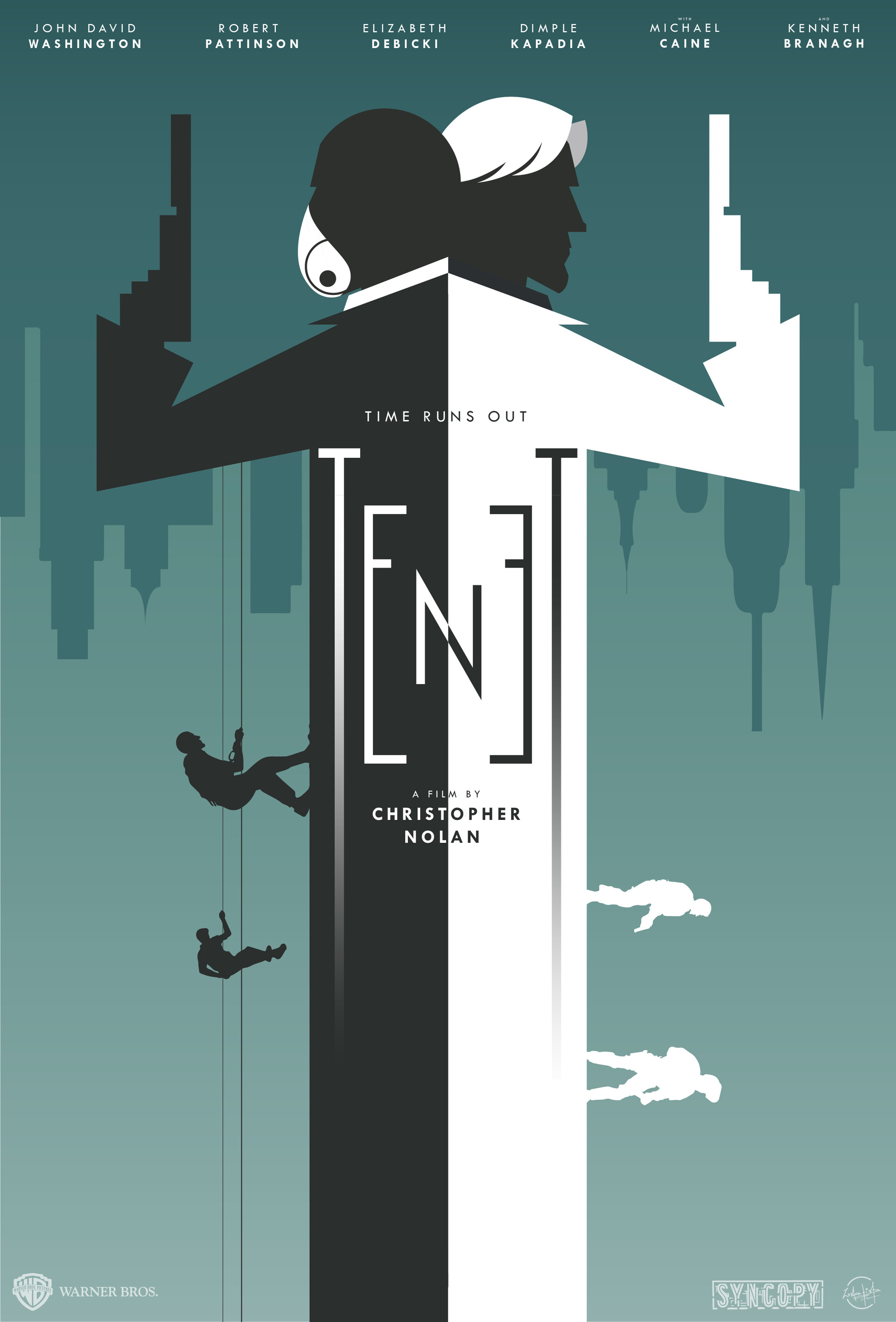This image is a promotional poster for the movie "TENET," directed by Christopher Nolan. The artwork illustrates a strikingly abstract and symbolic scene. Two men are depicted standing back-to-back; the man on the left wears a black suit that extends down to the bottom of the poster, with half of his face also in black, giving the illusion of wearing a mask. The man on the right dons a white suit, his face in black, with distinctive white hair. Both men are holding pistols pointed upwards as if poised for a duel. 

Additionally, there are silhouettes of men climbing on both sides of the duo—black silhouettes climbing up and white silhouettes descending down—adding layers of intrigue and motion. A notable element is the outline of an upside-down skyline at the top of the poster, shaded in blue, transitioning to a lighter blue towards the bottom. Centrally placed between the two men are the phrases "Time Runs Out" and "TENET," stylized with "TEN" written backwards in black within the white suit and in white within the black suit. At the top, the names "John David Washington" and "A Film by Christopher Nolan" prominently feature, tying the poster together.